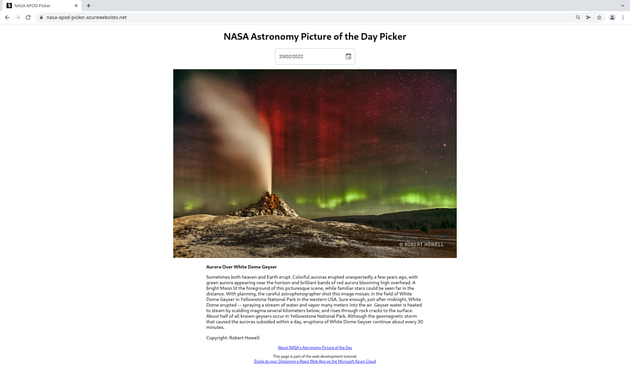This image is a blurry, pixelated screenshot of a web page that appears to be from NASA's "Astronomy Picture of the Day" feature. At the top of the screenshot, the title "NASA Astronomy Picture of the Day" can be discerned. Below the title, there is a text box and a URL bar at the top of the page, with some unreadable text on the browser tab.

The central part of the screenshot features a photograph that seems to depict a geyser or volcano emitting steam amidst a rocky terrain. In the background, there is a forest of trees, and the sky displays an atmospheric phenomenon similar to the northern lights with a blue and green neon haze.

Beneath the photograph, there is an unreadable title followed by a paragraph of text that is too small to decipher. At the very bottom of the screenshot, a blue hyperlink is visible.